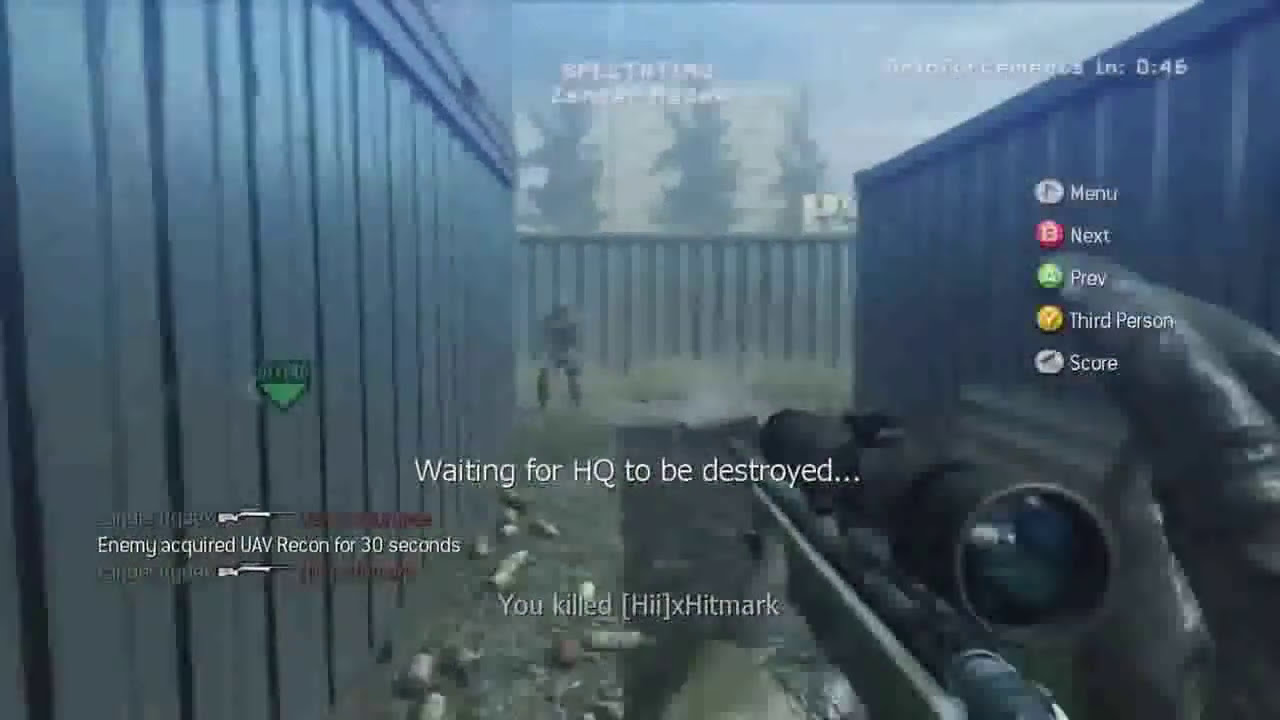This is a screenshot from a first-person shooter video game, possibly Call of Duty. The image is taken from the perspective of the player looking down the scope of a sniper rifle, with a gloved hand visible on the weapon. The screen is slightly pixelated and shows a warehouse-like area cluttered with garbage, with large dark gray shipping containers on the left and right and some trees and sky visible in the background. The scene is hazy and features smoke near the ground.

In the foreground, text in white reads, "Waiting for HQ to be destroyed... Below that, it states, "You killed [HII] X hitmark." Additionally, on the left side of the screen, there is a notification in white text that says, "Enemy acquired UAV recon for 30 seconds." The right side is framed by a navigation menu featuring colored buttons: a gray button labeled "Menu," a red B button for "Next," a green A button for "Prev," a yellow Y button for "Third Person," and a gray return button for "Score."

In the background, a soldier figure can be seen standing among the shipping containers, seemingly facing the player, accentuating the tension of the moment captured in this action-packed video game screenshot.